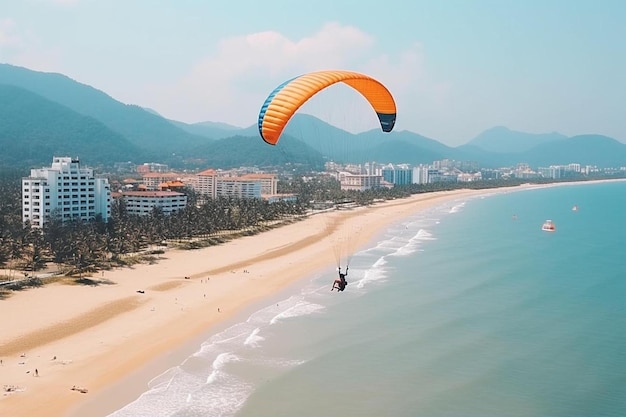In this detailed and realistic photograph, we see a person parasailing high above a scenic beach. The parasail is vividly colored with an orange canopy and blue trim. Below, the expansive ocean transitions from a light blue to a deeper shade, occupying the bottom right to the middle of the image. On the bottom left to the middle of the frame lies a sandy beach, a mix of yellowish-white and light beige tones. Viewed slightly from above, the beach is dotted with people strolling along its edge and interspersed with various ships in the water.

Adjacent to the beach, a series of palm trees add a tropical vibe, leading up to tall, multi-story buildings that resemble hotels and resorts. Beyond these structures, dark blue mountains and hills rise majestically against the lightly cloudy sky. The sky itself, a pale blue, contains only a wisp of a cloud, suggesting a mild, perhaps slightly stormy afternoon. The overall scene encapsulates a blend of natural beauty and human activity, making for a picturesque moment of adventure and tranquility.